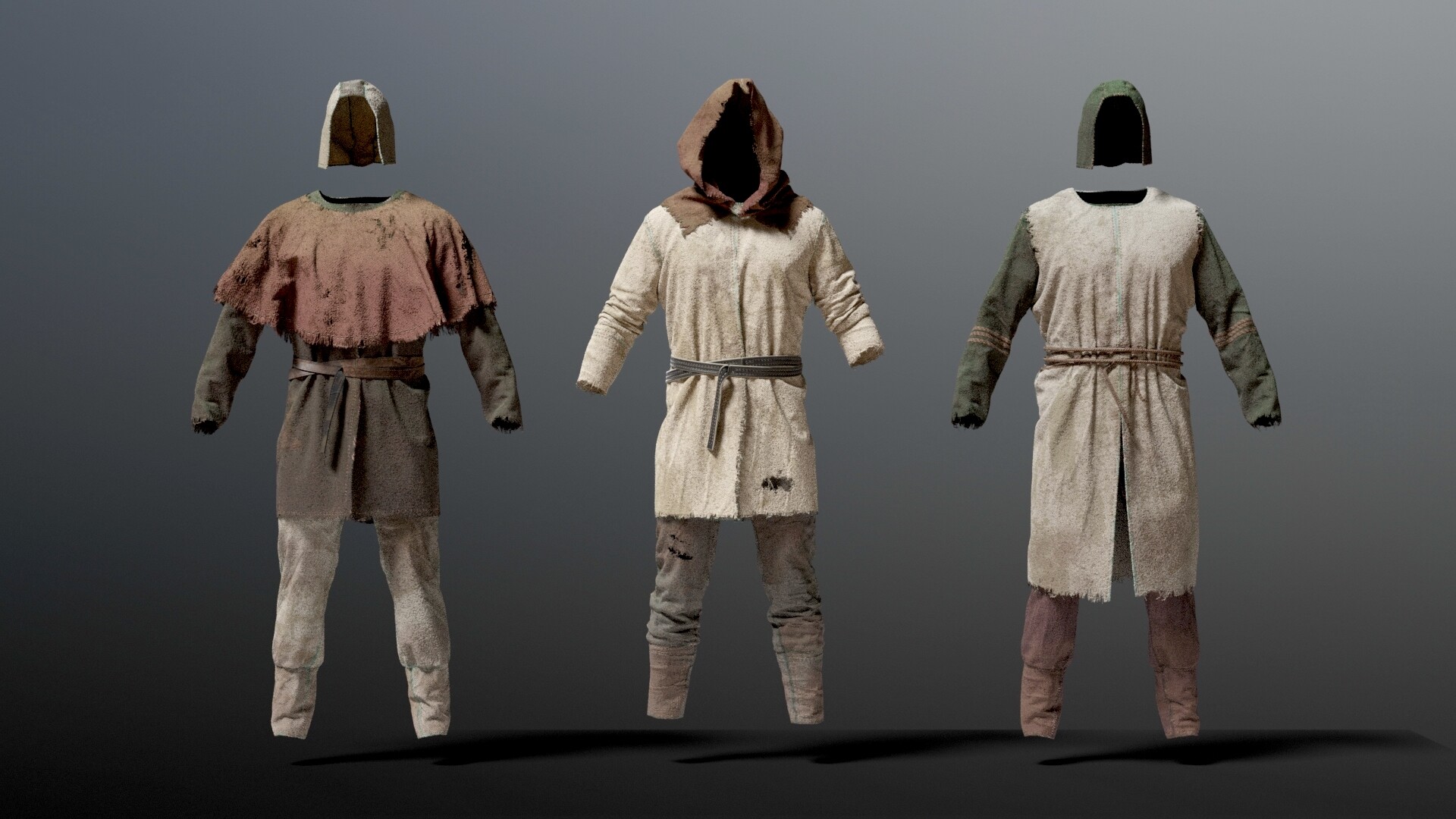The image showcases three digitally rendered outfits, each floating in midair as though invisible mannequins were wearing them. The background is a black to gray gradient, and shadows are cast below the garments, reinforcing the 3D effect. All three sets of clothing resemble medieval peasant attire, exhibiting a realistic texture and intricate details. 

The outfit on the left features a dull green tunic with an orange shoulder piece, accompanied by a white hood-like hat that hovers above. This ensemble includes white or gray pants and is cinched with a brown belt. Following this, the middle outfit consists of a white tunic tied with a blue sash, complemented by a brown hood and gray or brown pants. The final outfit on the right displays a white tunic with green sleeves and a green hood hovering above it. It is secured with a brown rope-like belt and paired with brown pants. Each costume gives off an aged, tattered vibe, reminiscent of clothing from ancient times.